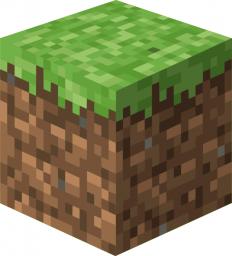This image showcases a pixelated block akin to those found in games like Roblox or Minecraft. The block is depicted from an isometric perspective, with its front turned slightly to the left corner of the image. This angle reveals three faces of the block: the top, the left side, and the front side. The top surface of the block is primarily green, with the green hue trickling down slightly over the edges of the other two visible sides. The body of the block is composed of a pixelated pattern featuring various shades of brown, ranging from light brown to dark brown. The distinct pixelated aesthetic of the block is emblematic of the iconic visual styles prevalent in these types of sandbox games.